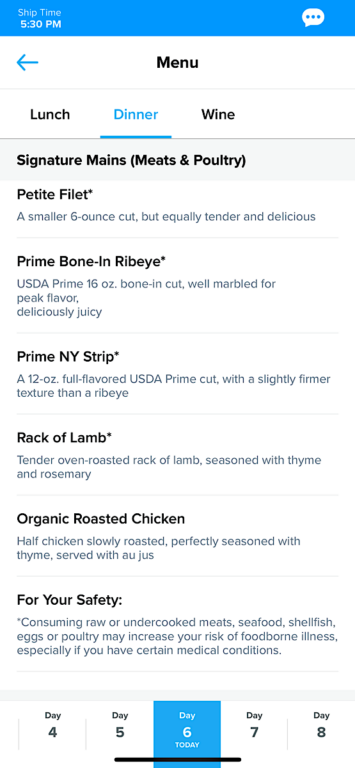In the image, we see a detailed view of a menu page, although the specific restaurant is not identified. In the top left-hand corner, the time is noted as 5:30 p.m. To its right, there is a messaging area, indicated by three dots that, when clicked, allow the user to write a message. Below this area, in bold black letters, the word "Menu" is prominently displayed.

The menu offers options for "Lunch," "Dinner," and "Wine," with the "Dinner" option currently selected and highlighted in blue. The dinner category breaks down further into sections labeled "Signature Mains," "Meat," and "Poultry." 

The menu items listed are as follows:
1. **Petit Filet:** A small six-ounce cut, equally tender and delicious.
2. **Prime Bone-In Ribeye:** USDA Prime 16-ounce bone-in cut, well-marbled for peak flavor, delicious and juicy.
3. **Prime New York Strip:** A 12-ounce full-flavored USDA Prime cut with a slightly firmer texture than a ribeye.
4. **Rack of Lamb:** Tender oven-roasted rack of lamb seasoned with thyme and rosemary.
5. **Organic Roasted Chicken:** Half chicken, slowly roasted and perfectly seasoned with thyme, served with au jus.

At the bottom, there's a health advisory warning: "For your safety, consuming raw or undercooked meats, seafood, shellfish, eggs, and poultry may increase your risk for foodborne illnesses, especially if you have certain medical conditions." Lastly, the date at the bottom of the page is the 6th, indicating that the current day is today according to the calendar.